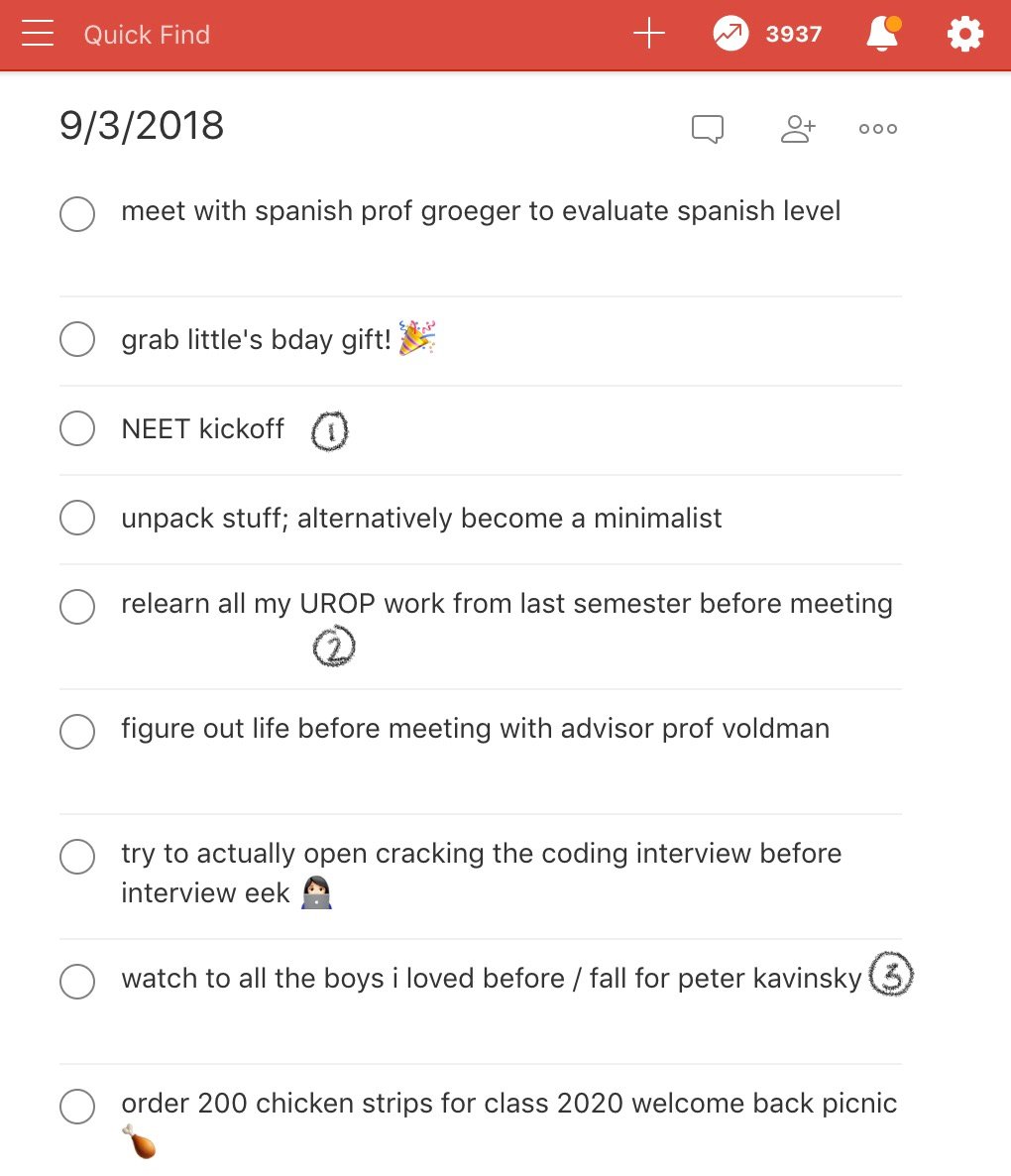Screenshot of QuickFind Website Interface

The screenshot depicts the QuickFind website, featuring a sleek and organized layout. The top of the screen is dominated by a bold red strip spanning from the left to the right edge. Within this strip, on the left side, there are three horizontal lines representing a menu icon, followed by the word "QuickFind," both in white. To the right of "QuickFind" is a white plus sign, a white circle containing a red upward arrow symbolizing a stock graph, the number 3937 in white, a notification bell with a small orange circle signifying an alert, and a gear icon presumably for settings.

Below the toolbar, the background switches to white with black text. The date "09/03/2018" is displayed prominently. On the far right, icons of a speech bubble and a person's head with a plus sign and three dots align horizontally.

The central portion comprises a detailed list, each item prefixed with a black-outlined circle on a white background, akin to bullet points:
1. "Meet with Spanish prof Gregor to evaluate Spanish level."
2. "Grab Little's B-Day gift" accompanied by a celebrations emoji with a party hat.
3. "Neat kickoff!" marked as highly important with a handmade pencil circle and the number one.
4. "Unpack stuff. Alternatively become a minimalist" displaying a bit of humor.
5. "Relearn all of my UROP work from last semester before meeting" circled with a two inside.
6. "Figure out life before meeting with advisor prof Valdman."
7. "Try to actually open 'Cracking the Coding Interview' before interview eek" illustrated with a picture of a woman using a laptop.
8. "'To All the Boys I've Loved Before' for Peter Kavinsky" circled with a hand-drawn number three.
9. "Order 200 chicken strips for class 2020 welcome back picnic" ending with a chicken drumstick emoji.

Overall, the screenshot encapsulates a user-friendly interface combining functionality with a touch of humor and personalization.